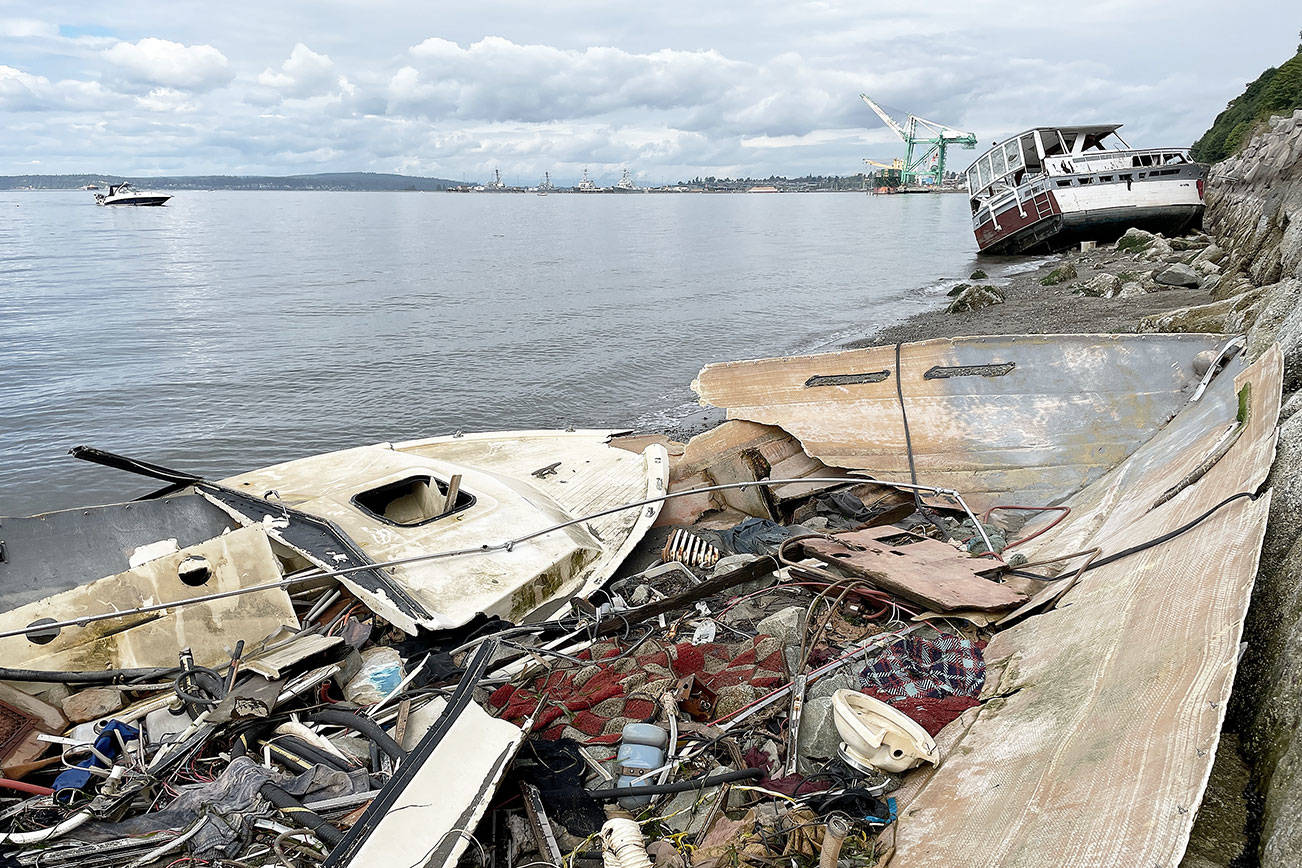The image depicts a cloudy day along the shoreline of a large, still body of water. In the foreground, a cliff with gray rocks and patches of green vegetation is visible on the right side of the image. Strewn across the rocky shore are remnants of wrecked boats, including a small disintegrated brown canoe and a partially intact white and red vessel. Litter such as blankets, wire rods, and boat parts are scattered around, highlighting the aftermath of multiple shipwrecks. Against the backdrop, a sailboat floats in the calm, gray water, and further out, hills are faintly visible beneath a sky filled with light gray clouds. In the distance, a green and white crane-like heavy equipment can be seen, adding a hint of industrial presence to the otherwise desolate scene.